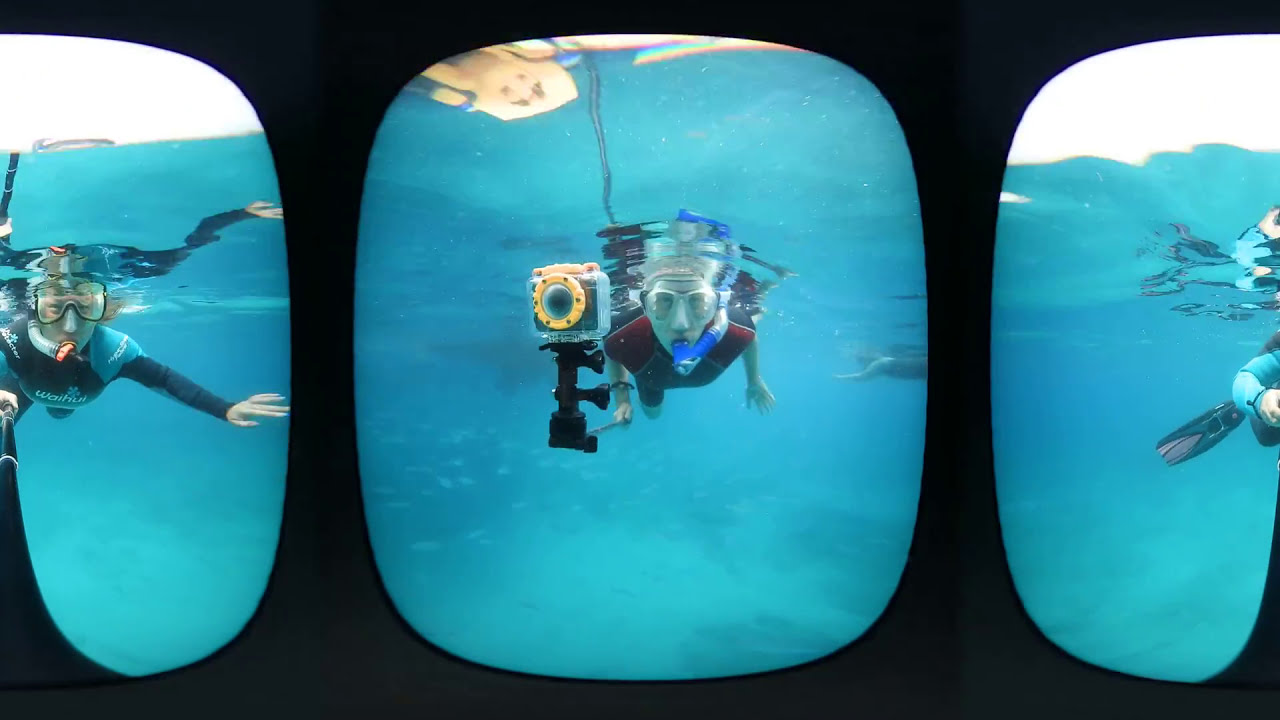The image features three sections viewed as if looking through multiple submarine windows against a solid black background. Each section is shaped like a vertically rounded rectangle, creating the effect of portholes. In the left section, half of a window is filled with a light blue body of water where a snorkeler, wearing a black wetsuit with blue accents and a white snorkel, faces the camera. This diver holds a slightly bent camera pole with a black mount. The middle section, displaying an entire window, showcases another diver directly facing the viewer, wearing a red short-sleeve wetsuit and blue snorkel. This diver's right hand grips a camera mounted on a black handle with a yellow casing around the lens. Lastly, the right section shows only half of a window, capturing a partial view of water with an arm and the back scuba fin of another diver. The background suggests an indoor setting, possibly from the perspective of someone inside a submarine, with the contrasts in colors highlighting the light blue water, black wetsuits, and camera equipment.